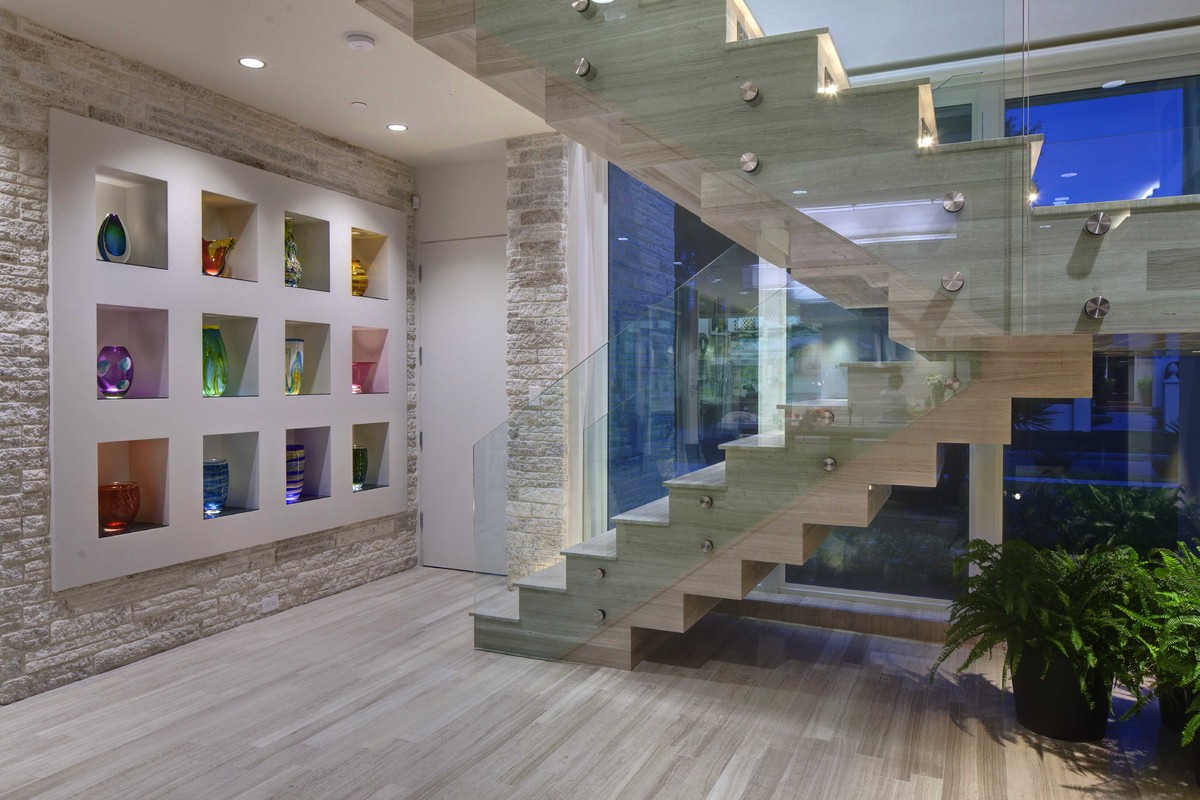The image captures the interior of a stylish and modern house or business space. The central focus is a sleek staircase with glass railings, allowing a clear view of its contemporary architectural design. Just beneath the staircase are two lush green plants in black pots. Behind the staircase, there's a large glass window revealing a blue-lit room, suggesting it's late at night. On the left side of the staircase, there's a door leading to the room behind the glass. Adjacent to this door is a built-in white cabinet showcasing an array of colorful vases—each compartment illuminated to highlight the distinct hues of blue, orange, green, purple, red, light blue, dark purple, pink, black, and yellow. This scene sits within a softly lit space, adding to the elegant ambience.